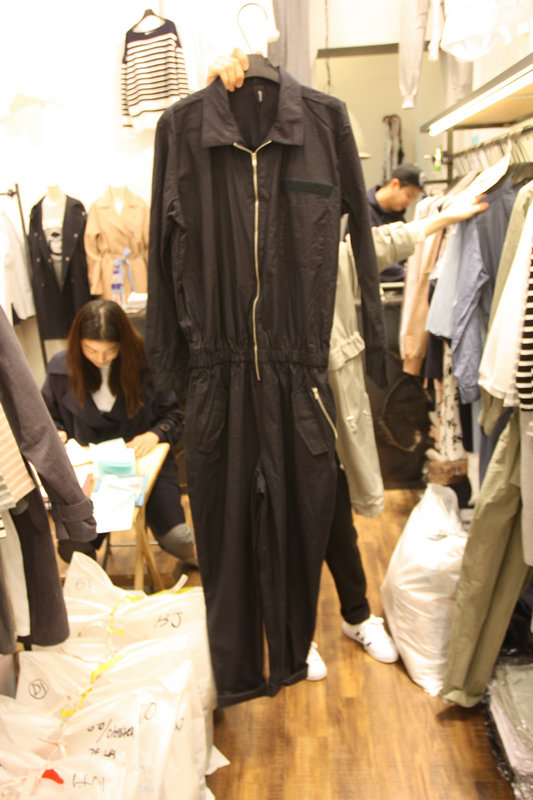This color photo captures a bustling clothing store environment with a central focus on a black jumpsuit being held up by an unseen person, their hand visible at the top left. The jumpsuit, characterized by its wrinkly texture, features a silver zipper running down the front and a cinched waist, along with pant pockets embellished with zipper detailing. It hangs on a black hanger, grounding the scene amidst a vibrant background filled with various shop elements.

On the right, multiple clothes racks display a diverse array of garments, including a mannequin donning a black jacket over a white shirt and another in a tan trench coat. Additional clothes are visible, including a black-and-white striped shirt hanging high in the background. 

To the left, just partially visible, another rack of clothes and bustling store activities draw attention. A woman with long brown hair wearing a black jacket, gray pants, and a white undershirt is working on paperwork, her hands moving through documents stacked around her. Nearby, a line of white plastic bags with hard-to-read black lettering is on the ground.

Seated behind these bags is another woman, engrossed in something off-camera, while a man in the background, wearing a black hat with a white logo and a dark blue hoodie, adds a casual element to the scene. Completing the tableau, a light-skinned woman in a gray trench coat reaches out to touch a dark blue dress shirt, with her white shoes and black pants peeking from behind a black tracksuit.

Overall, the image encapsulates the dynamic and detailed setting of a busy clothing store, highlighting both the central jumpsuit and the myriad activities and individuals around it.